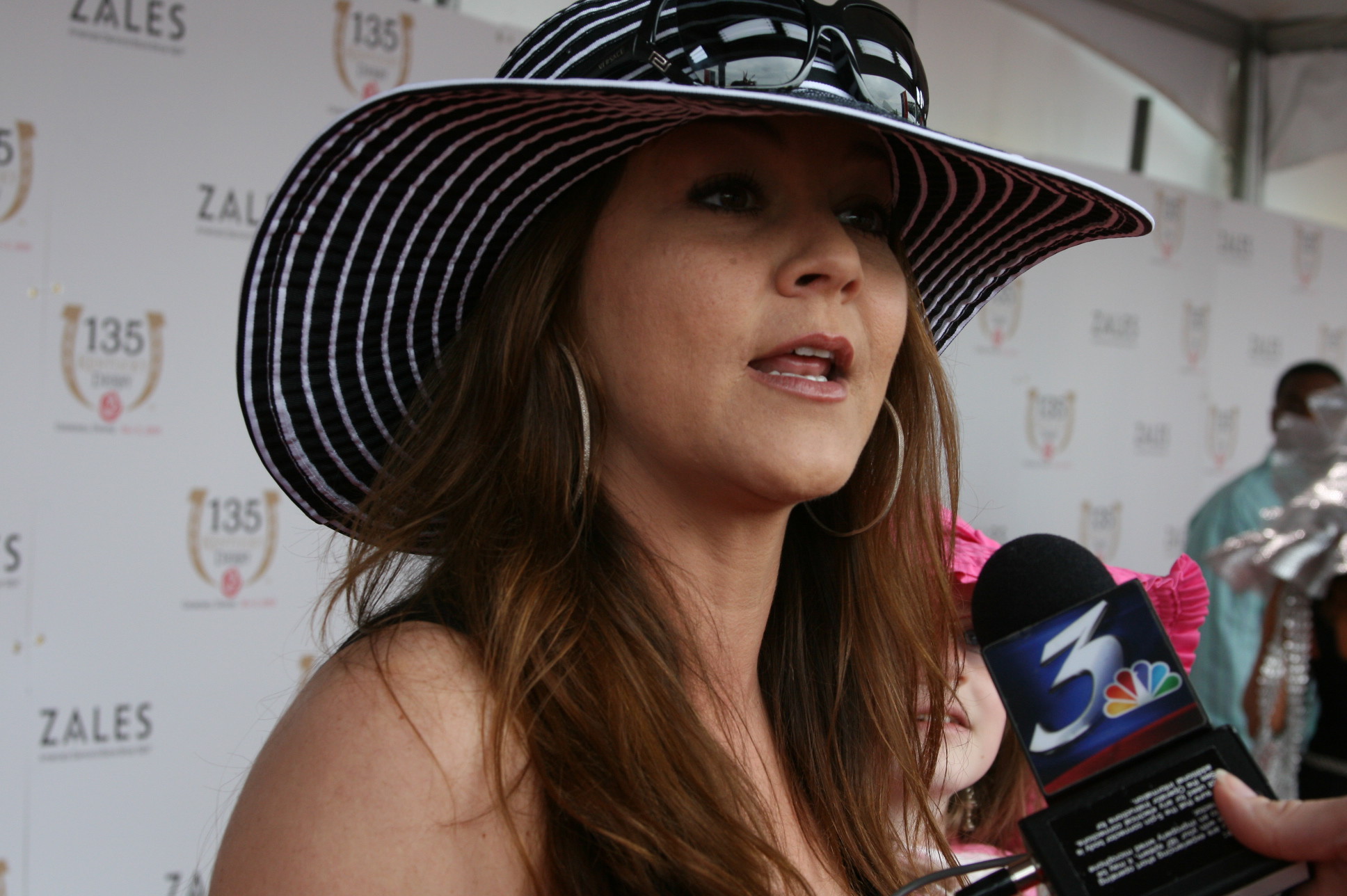In the image, a young woman, possibly in her 30s or 40s, is captured mid-conversation while being interviewed. She sports a black and white striped sun hat with black sunglasses perched on top. Her long brown hair flows beneath the hat, and she accessorizes with large hoop earrings. A hand holding a microphone numbered '3', adorned with a colorful TV logo, is positioned close to her face. The setting appears to be a public event or fashion show, featuring a white panel backdrop with various writings and company logos, including "ZEUS" and the number "135". Below the woman, there is another individual wearing a pink hat, and a younger girl, possibly her daughter due to their similar appearance, stands next to her. The scene is lively with people in costumes visible to the right.